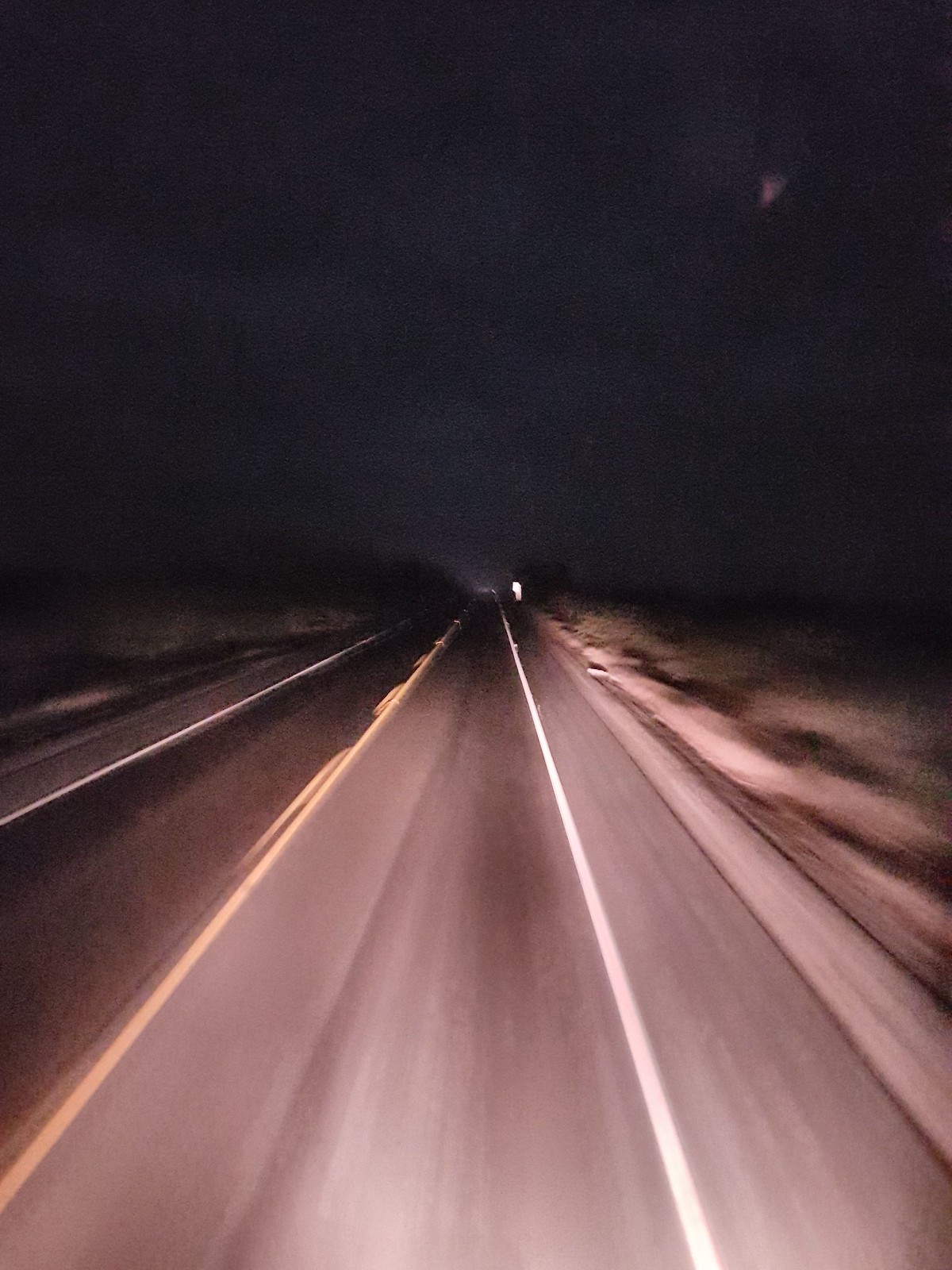In this nighttime photograph, slightly blurred as if captured from a moving vehicle, a two-lane road stretches out ahead. The sides of the road blur into a monotony of flat grass, complemented by distant trees slightly off the road. The asphalt, illuminated by the vehicle's headlights, reveals a white line marking the right edge and a yellow line dividing the lanes. In the far distance, the headlights illuminate an approaching road sign. The sky above is an impenetrable black, and far off, the faint lights of another vehicle are just visible, adding a sense of depth and solitude to the scene.